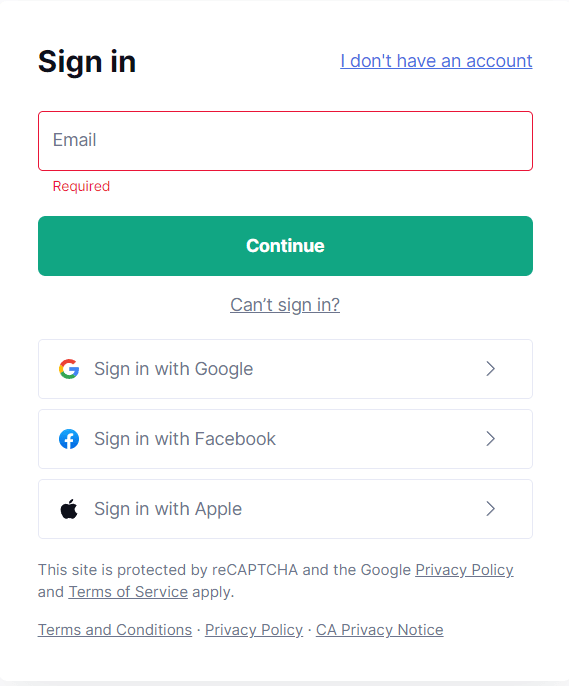The screenshot displays a simple login page with a white background that facilitates user authentication through several options. At the very top left corner, there is a bold, black "Sign In" text, while the top right corner features a blue, underlined link stating "I don't have an account," indicating it is clickable for new users.

Beneath these elements is a red-bordered input box labeled "Email" in black text, where users are required to enter their email addresses. The box currently shows the placeholder text "Required," indicating no email has been entered yet. Below the email input box is a prominent green button labeled "Continue," suggesting the next step in the login process.

Further down, there is a black text link that reads "Can't sign in," providing help for users experiencing login issues. Below this link are three additional buttons for alternative sign-in methods: "Sign in with Google," "Sign in with Facebook," and "Sign in with Apple." The "Sign in with Google" button is marked with a greater-than sign (">"), hinting at a possible dropdown or additional options.

At the bottom of the page, informational text is displayed indicating that the site is protected by reCAPTCHA, followed by links to the "Terms and Conditions," "Privacy Policy," and "CA Privacy Policy," allowing users to review the site's policies. The page concludes with a subtle gray border at the very bottom.